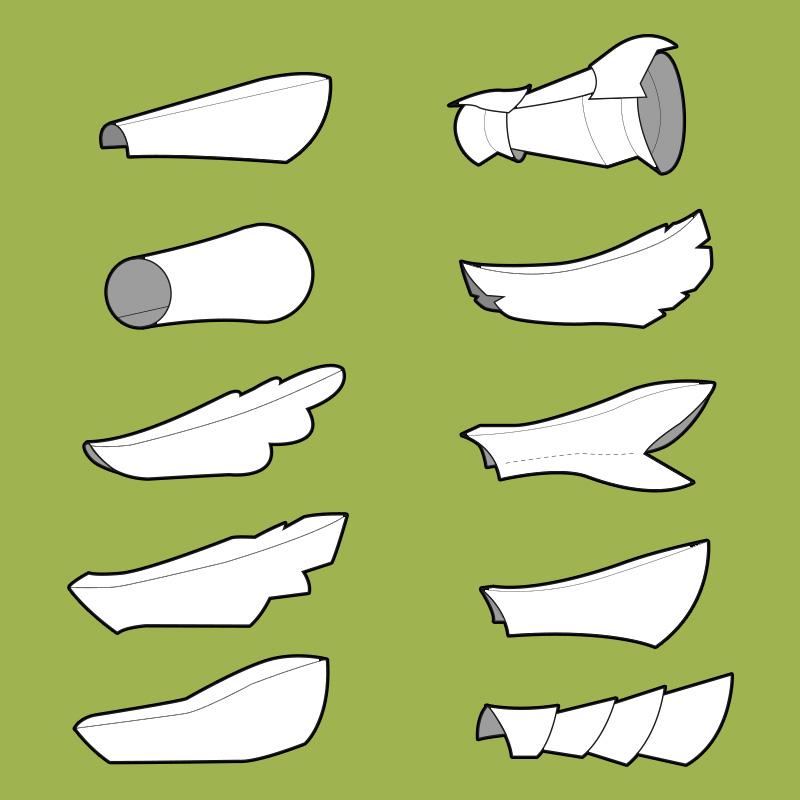This artwork features an olive green background adorned with ten intricately detailed white illustrations. These objects, outlined in thick black lines and accented with gray shading, are symmetrically arranged in two vertical rows of five on the left and right sides. Each shape resembles a piece of armor or a decorative element, such as spauldrons, wrist guards, and gloves. Some shapes resemble cuffs, sleeves, or even tails, evoking imagery of leaves, feathers, oak leaves, paws, and insectoid, articulated arms. The illustrations are detailed with black dotted seams, adding to their intricate design. Notably, two shapes are complete tubes, while the others appear as if tubes were cut in half and artistically altered.